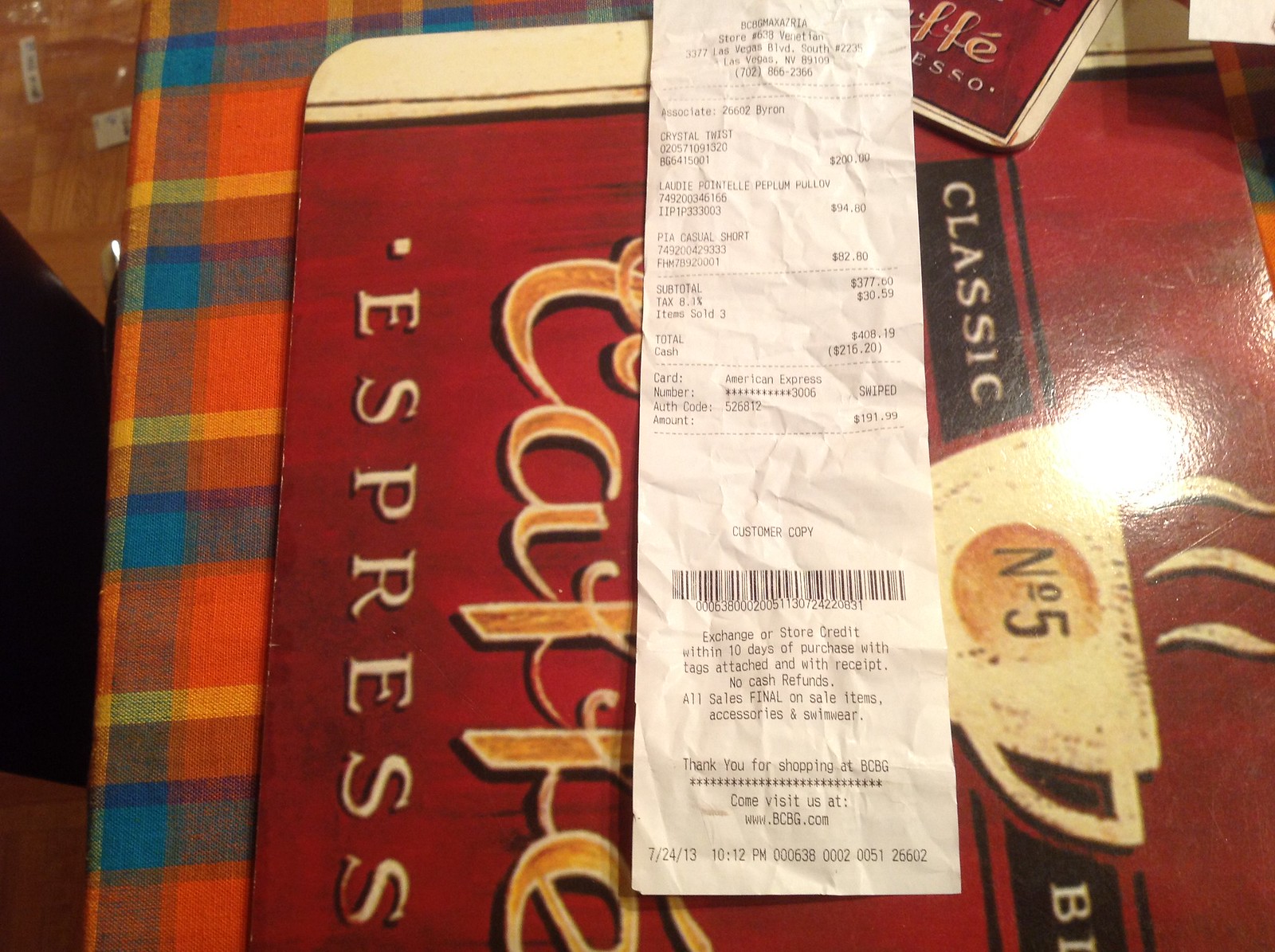This is a detailed close-up photograph of a white, crumpled receipt placed atop what appears to be a vividly designed table setting. The receipt, which is notably wrinkled and improperly folded, has its top text rendered illegible, interrupted by two dotted lines. Below the unreadable segment, the receipt lists several products in black ink on the left, with corresponding prices on the right—a line item that might read "crystal twist" with an unclear price, possibly 200. The subtotal and tax are mentioned but equally blurred. The total is documented as $408.19, with a cash payment of $216.20. A barcode and long string of numbers denote it as a "customer copy," followed by a store policy section proclaiming "exchange or store credit." The bottom notes, "Thank you for shopping at BCBG. Come visit us at www.bcbg.com," along with the date, 7-24-13, and time, 10:12 PM, plus a serial number 000-638 and an additional sequence of numbers.

The receipt rests on top of a sign featuring intricate design elements—a depiction of a white coffee cup with dark brown splotches, circled by milk chocolate brown and dark chocolate brown numbers, an "N" with a tiny "0," all set against a maroon red background. The sign reads "classic" and partially visible "B" followed by indistinct text. Curyl-Q letters spell "coffee" in orange bordered by white, with "espresso" being partially cut off.

This entire arrangement is laid on a plaid tablecloth boasting an array of colors: red, maroon, dark blue, dark gray, orange, and olive green. The receipt is centered, surrounded by hints of a table mat showing the text "classic number five coffee express" against a textured red backdrop. To the left, a glimpse of the floor is visible, suggesting the setting is within a home, richly adorned with a busy table showcasing this detailed receipt-focused tableau.